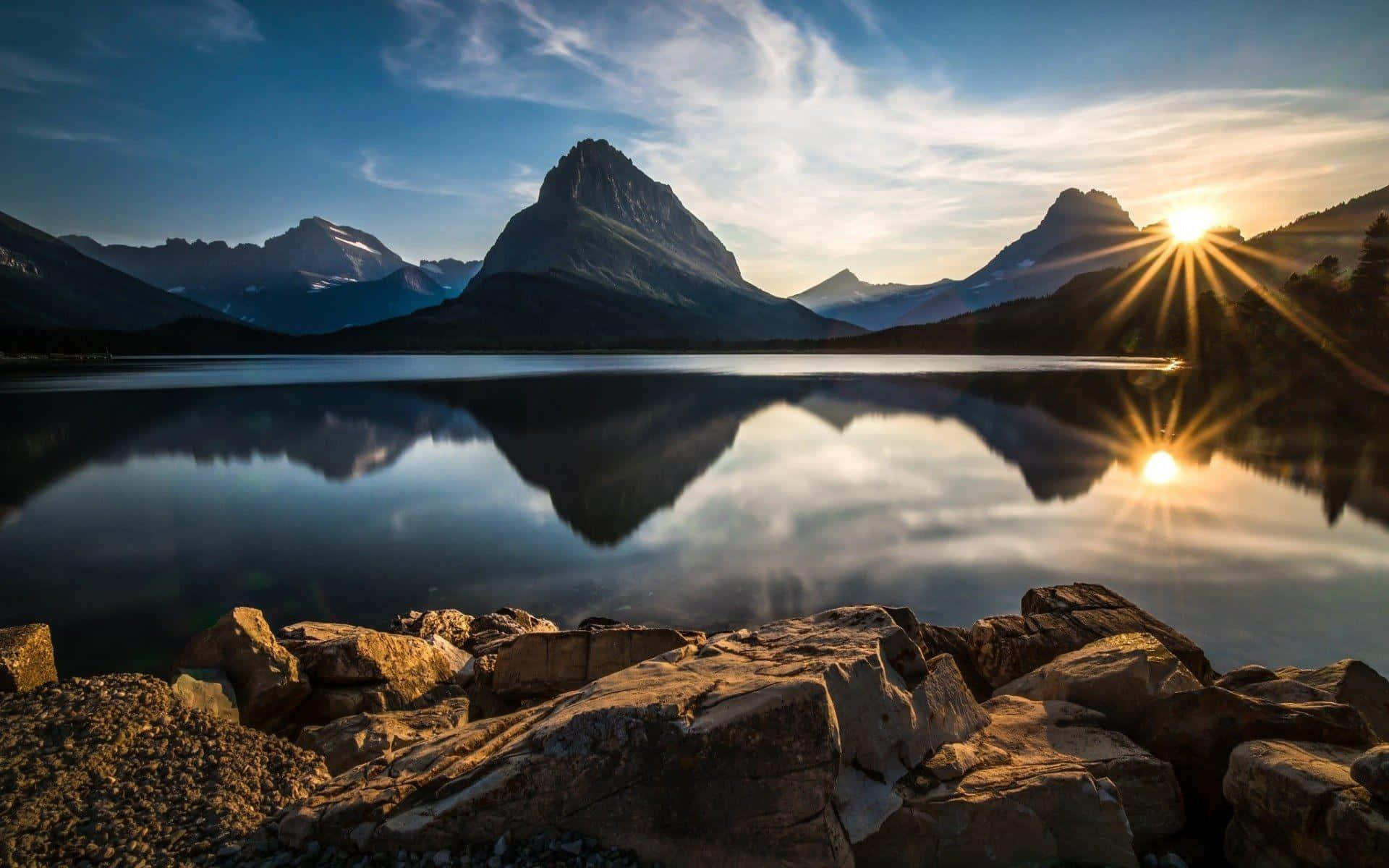In this photograph, a serene lake stretches out before a grand mountain range, with the sun either rising or setting behind the peaks. The towering mountains, primarily brown with occasional white snow caps, dominate the background. The still waters of the lake perfectly reflect the majestic mountains and the vibrant colors of the sunrise or sunset. The sky above is a serene blue, dotted with scattered clouds. The sun's hues of yellow and orange illuminate the scene, casting a warm glow. In the foreground, a rocky shoreline composed of brownish-gray rocks and some gravel leads the viewer's eye towards the lake. To the right, a faint tree line adds a touch of green to this natural tableau, completing a breathtaking landscape scene.